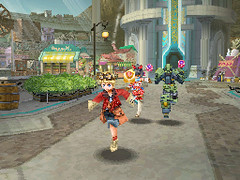This image, a screenshot from a video game, depicts a vividly animated scene with three colorful, long-legged characters resembling Japanese anime, running along a gray pathway. The characters cast small, circular shadows beneath them. The left side of the background is dominated by a blue sky transitioning into a tan building with a prominent, neon-lit doorway featuring yellow and blue lights that outline the entrance. In front of this building, a silver, rounded structure adds to the futuristic aesthetic. The right side presents a whimsical, pink building with a ground-level windmill-like structure. The scene also features elements of a fantastical world, including candy cane-striped awnings, a yellow and white canopy, green flowers in a flower bed, and overall vibrant greenery. The image imbues a sense of whimsy and adventure with its mix of futuristic and fantastical elements.